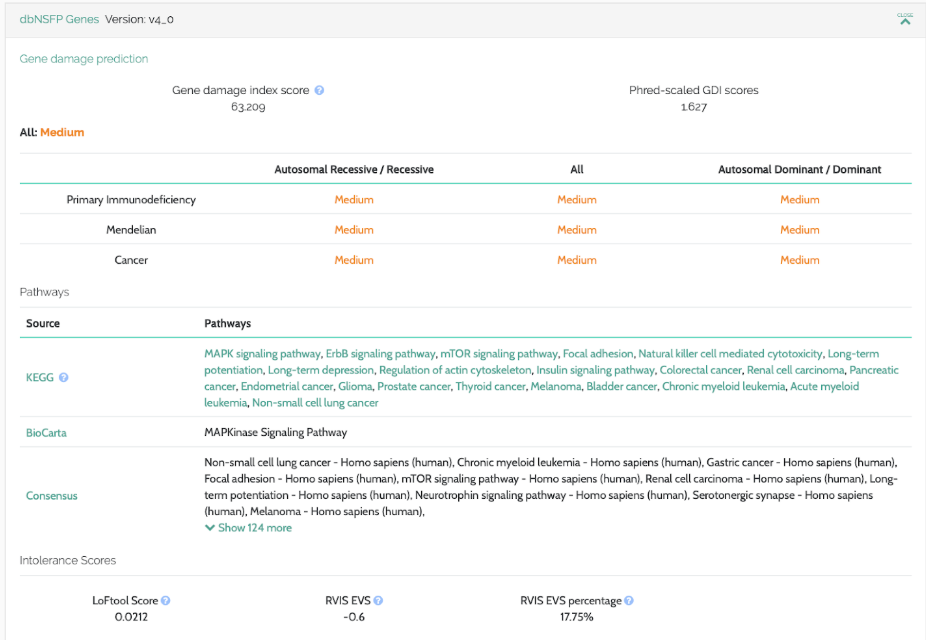Screenshot of the DB NSFP Genes Interface, Version v4.0

The screenshot, captured in landscape mode, features the DB NSFP Genes interface, version 4.0. The top left corner showcases a gray stripe bearing the text "DB NSFP GENES version v4.0". The text "DB NSFP GENES" is rendered in teal, while "version v4.0" is in black. On the upper right-hand corner, a prominent green "Close" button is visible. 

Beneath the gray stripe, the rest of the interface has a white background. The upper left section is highlighted in green with the title "Gene Damage Prediction". Directly below this title, a row begins with "Gene Damage Index Score" followed by a numerical value inside a blue circle, displaying "63.209". Adjacent to this, the "PHRED scaled GDI score" is noted as "1.627".

Proceeding to the next section, the text "ALL" is capitalized on the left, with the term "medium" in orange beside it. Below is a detailed chart. The columns are labeled as follows from left to right: "Primary Immunodeficiency," "Mendelian," and "Cancer." The rows beneath these headings display the categorization of genetic conditions: "Autosomal Recessive," "Medium," "Medium," "Medium"; "All," "Medium," "Medium," "Medium"; "Autosomal Dominant," "Medium," "Medium," "Medium."

Further down, another section is dedicated to pathways, with the topmost columns labeled "Source" and "Pathways." The sources listed include "KEGG," "Biocarta," and "Consensus."

At the bottom of the screenshot, there is a segment labeled "Intolerance Scores." Due to the limited view of the screenshot, details of this section are less clear.